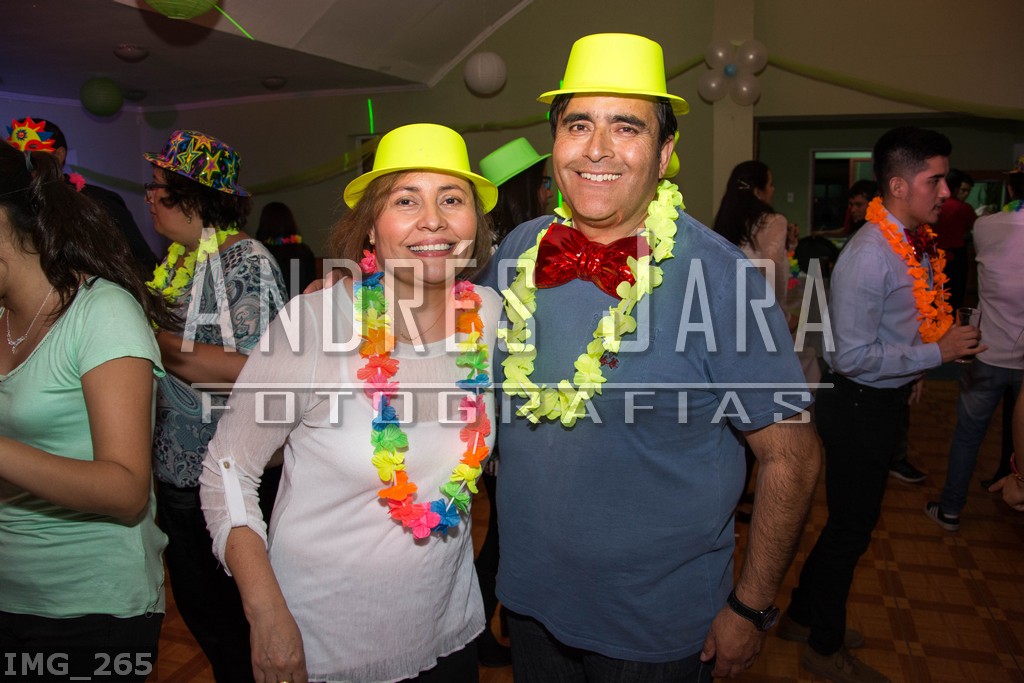In the center of this lively party scene, a man and woman take center stage, directly engaging the camera with cheerful expressions. The man, somewhat older with darker skin and black hair, is adorned in a festive outfit featuring a neon yellow top hat, a large red bow tie, and a green plastic flower garland around his neck. He’s wearing a blue shirt and a wristwatch. Beside him stands a middle-aged woman with brown hair, clad in a light pink long-sleeve top, also sporting a neon-colored hat and a vibrant, multicolored flower garland.

Surrounding the duo is a bustling party atmosphere filled with numerous adults, both male and female, clad in varied attire from formals to casuals. Many guests wear similar plastic flower garlands, indicating a possible theme like a luau. The background reveals a spacious, moderately lit hall, possibly a decorated house or a conference room, adorned with balloons, lights, and patterned flooring. People can be seen mingling, holding drinks, and moving about, adding to the lively ambiance.

Over the image, a semi-transparent white watermark reads "Andreas Jara, Fotografias," indicating a professional touch to the photograph. Additional details such as walls, pillars, and doors frame the scene, with the watermark IMG_265 subtly present at the bottom corners.

Overall, this image captures a vibrant celebration with a colorful and joyous atmosphere, central to which are the festively dressed man and woman, posing happily for the camera amidst the bustling crowd.